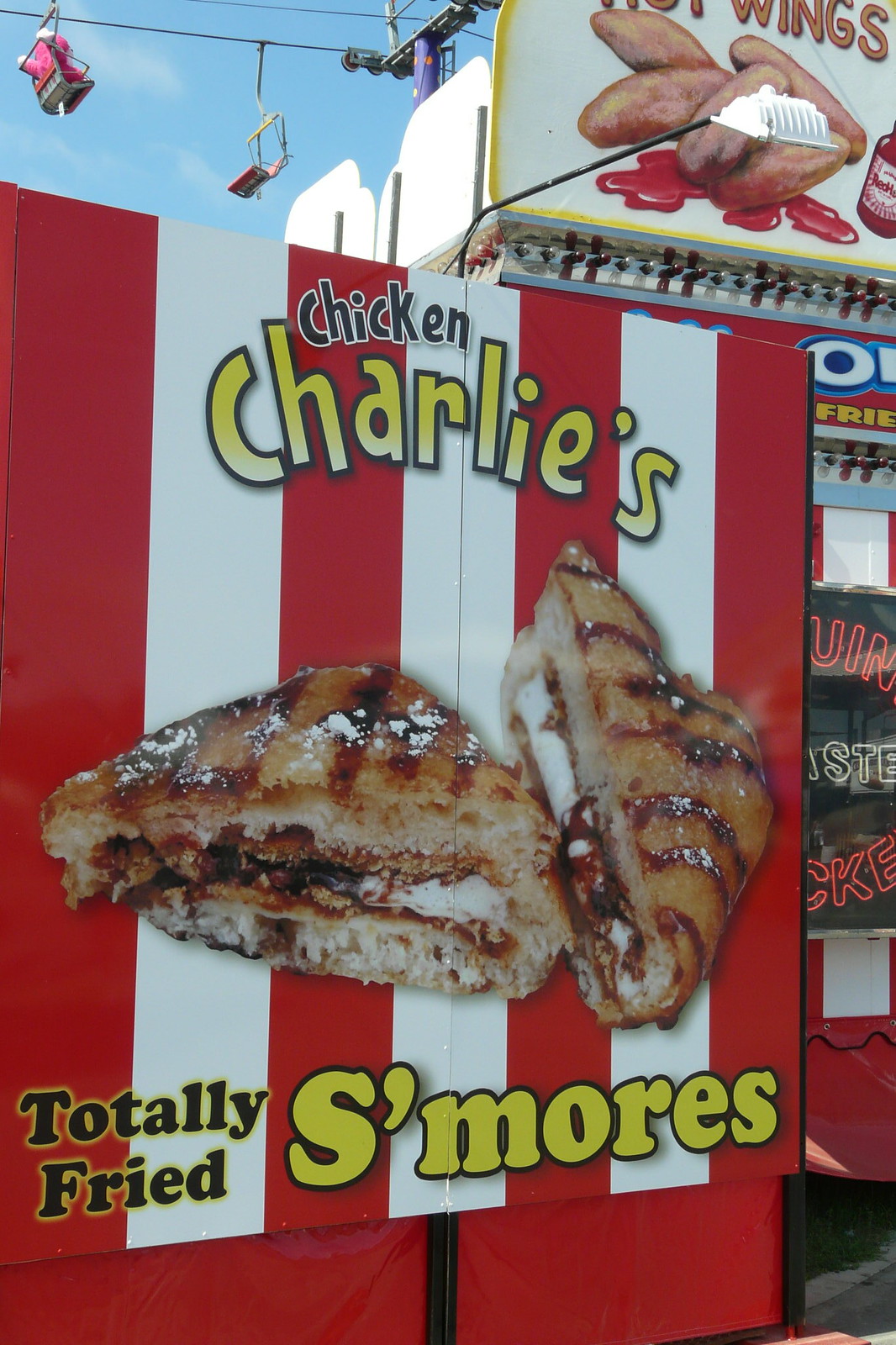The picture showcases a vibrant advertisement for Chicken Charlie's, prominently featuring their Totally Fried S'mores. The backdrop of the photo suggests a fair setting, indicated by the blue skies and a ski lift visible above the signage. The central sign, adorned with striking vertical red and white stripes, has bold lettering: "Chicken" in black, "Charlie's" in yellow, and "Totally Fried S'mores" in a contrasting mix of yellow and black. The delectable image of fried s'mores, dusted with powdered sugar, takes center stage on the sign. To the right, a booth with a billboard displaying chicken in red sauce and a partially visible red and white neon sign adds to the festive atmosphere. The fairground's pavement is faintly visible in the bottom right corner, further grounding the lively scene.